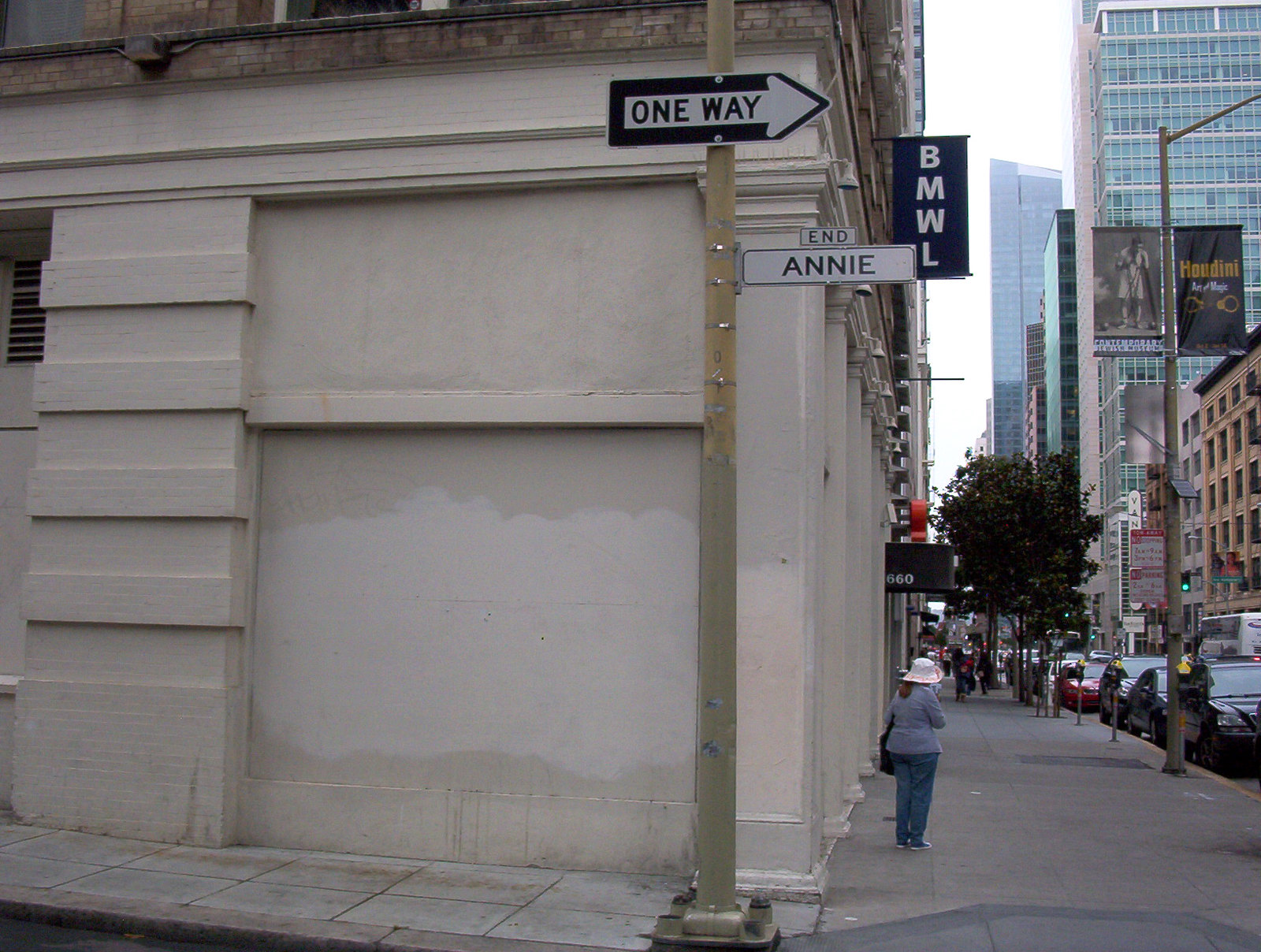The image showcases a bustling city street corner dominated by a large, tan-colored concrete building with ornate brickwork on its upper portion. The building features a sidewalk made of cinder blocks that curves around its front, where a tall metal signpost stands. The signpost displays a black and white one-way sign pointing to the right, with a secondary sign beneath it reading "End Annie." To the right of the image, the street extends with several parked cars and modern skyscrapers featuring glass windows. Among the pedestrians, a prominent figure in the foreground wears a white and pink hat, a gray jacket, and blue pants, while other people can be seen further down the sidewalk. The scene is enriched by the presence of trees and two advertisement banners. Additionally, a blue banner with the letters "BMWL" is affixed to the building, adding a splash of color to the urban landscape.